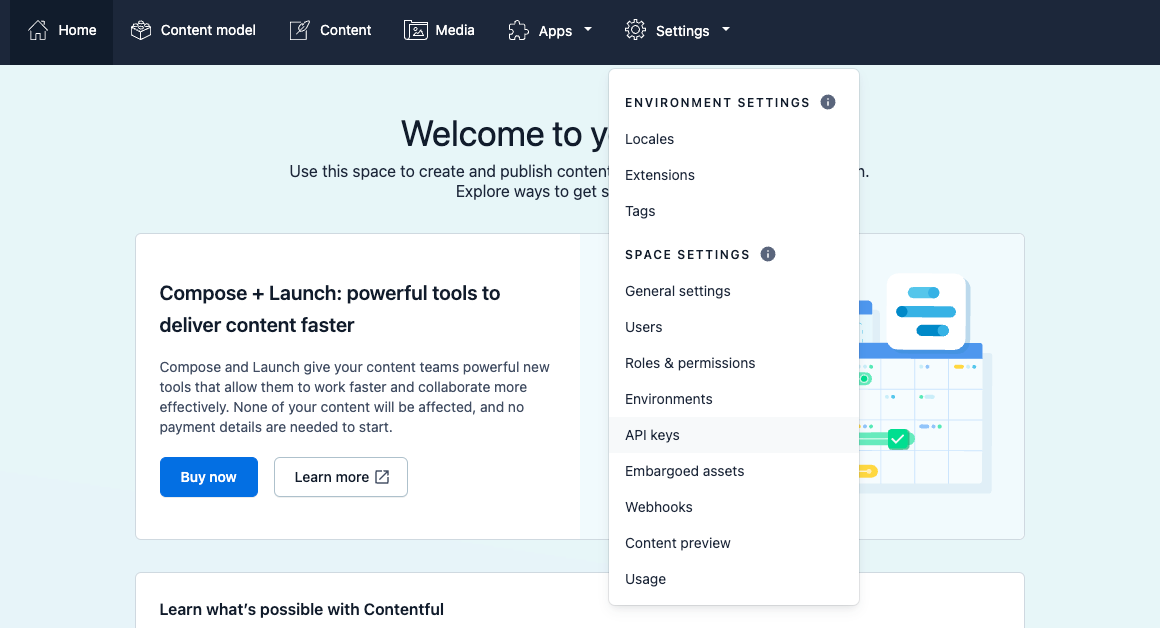The image features a black rectangular banner spanning across the top. In the upper left-hand corner of this banner, there is a white outline of a house icon accompanied by the word "Home" in white. Next to it, a white cube icon appears with the label "Content Model." Following this, an icon resembling a feather on a piece of paper is marked with the word "Content" in white. Another icon that looks like a puzzle piece is labeled "App" in white. Adjacent to this, there is a white gear icon labeled "Settings."

The background transitions to a light blue color below the banner. In black text, the phrase "Welcome to" is displayed, followed by text that partially reads "use this space to create and publish content," though part of it is obscured by a pop-up window. Another partially visible line says "Explore ways to get," but a pop-up obstructs the completion of this sentence. 

The white pop-up window lists various settings and tools in black text, including "Environment Settings," "Locales," "Extension," "Tags," "Space Settings," "General Settings," "Users," "Roles," and "Permissions." Additional options displayed in black text are "Environments," "API Keys" (highlighted in gray), "Embargoed Assets," "Webhooks," "Content Preview," and "Usage."

Beneath the pop-up, there is a white rectangular background with black text that reads, "Compose + Launch... powerful tools to deliver content faster. Compose and Launch gives your teams powerful new tools that allow them to work faster and collaborate more effectively. None of your content will be affected, and no payment details are needed to start." 

Two buttons are presented on the left side below this text. One button has a blue background with the words "Buy Now" in white, and the other button has a blue outline with "Learn More" written in black text in the middle.